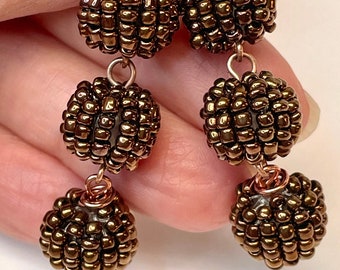This indoor photograph features a close-up view of jewelry, possibly earrings, captured against a slightly off-white background. The background has a subtle gradient, with an orangish tone along the right side and a whiter, shadowed area beneath. Dominating the frame are three fingers and part of a thumb of a Caucasian woman's hand, positioned in the upper right corner. The hand delicately holds two rows of intricate bead clusters. Each row consists of three globe-shaped clusters, each adorned with numerous platinum-colored beads, giving them a blackberry-like appearance. These clusters are connected by short gold rings, adding an antique charm to the piece. The jewelry exudes a vintage elegance, making it unclear whether they serve as earrings, part of a necklace, or some decorative accessory. The image is cropped to a small, almost square dimension, approximately two inches wide and an inch and a half high, emphasizing the delicate craftsmanship of the bead clusters and gold rings.